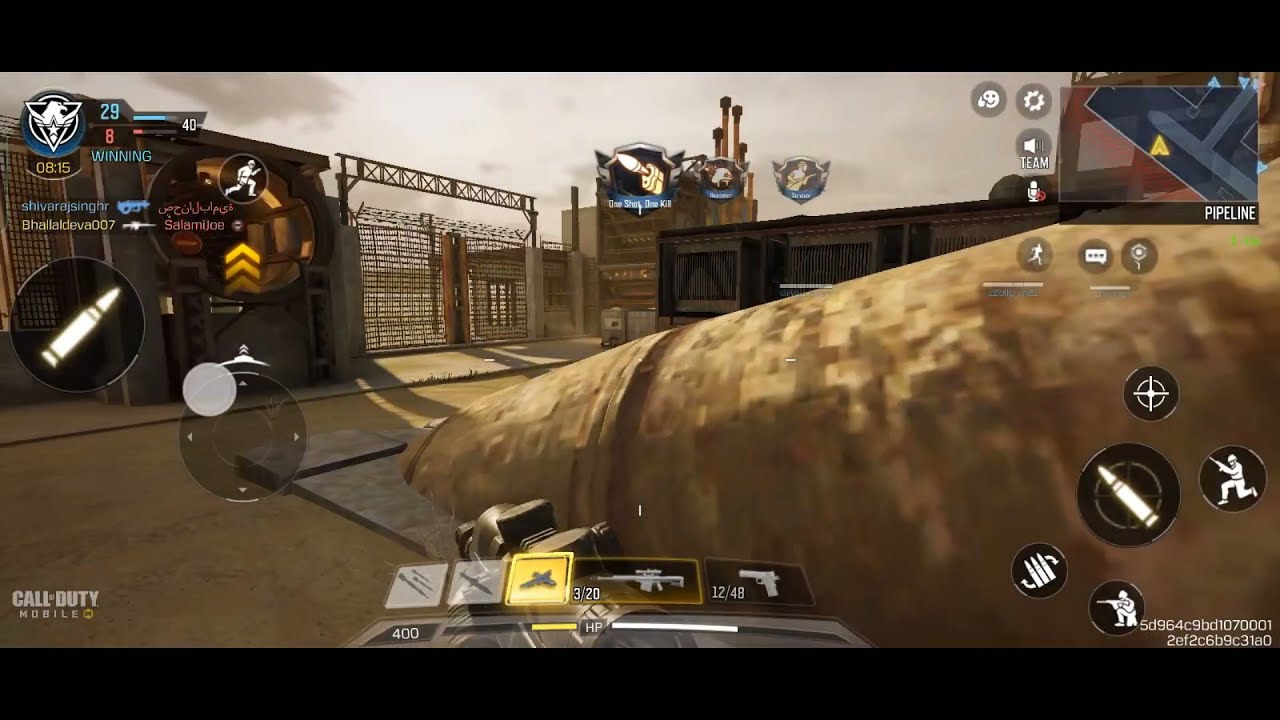The image is a detailed screenshot from the video game **Call of Duty Mobile**, capturing the interface of a first-person shooter perspective. Featured prominently in the lower left corner is the game title, "Call of Duty Mobile." The scene is set in what appears to be an industrial courtyard, characterized by dull gray skies.

In the center foreground of the image, there is a large, russet-brown boulder resembling a potato growing out of the ground, which the player is using for cover. This outdoor setting includes a sizable metal fence in the background, and an industrial factory with smokestacks.

On the screen, various gameplay icons and controls are visible, crucial for in-game actions. The right-hand side of the screen displays several notable icons: one of a bullet, a crouching man with a weapon, an aiming target, and a kneeling figure. Additional icons include an ammo count and gun switch options.

In the upper right-hand corner, a mini-map with a yellow arrow indicates the player's position within the game world. Three icons in the middle provide details on the teammates’ locations. The upper right corner also displays the game status, noting "29," indicating the score, alongside a bee icon and gun icons. The bottom right corner includes various logos, such as a scope, target, bullet, and a kneeling figure with a gun further emphasizing the militaristic and tactical nature of the game.

Overall, the image effectively captures the immersive, detail-rich interface of Call of Duty Mobile, highlighting the combination of strategic elements and industrial setting.